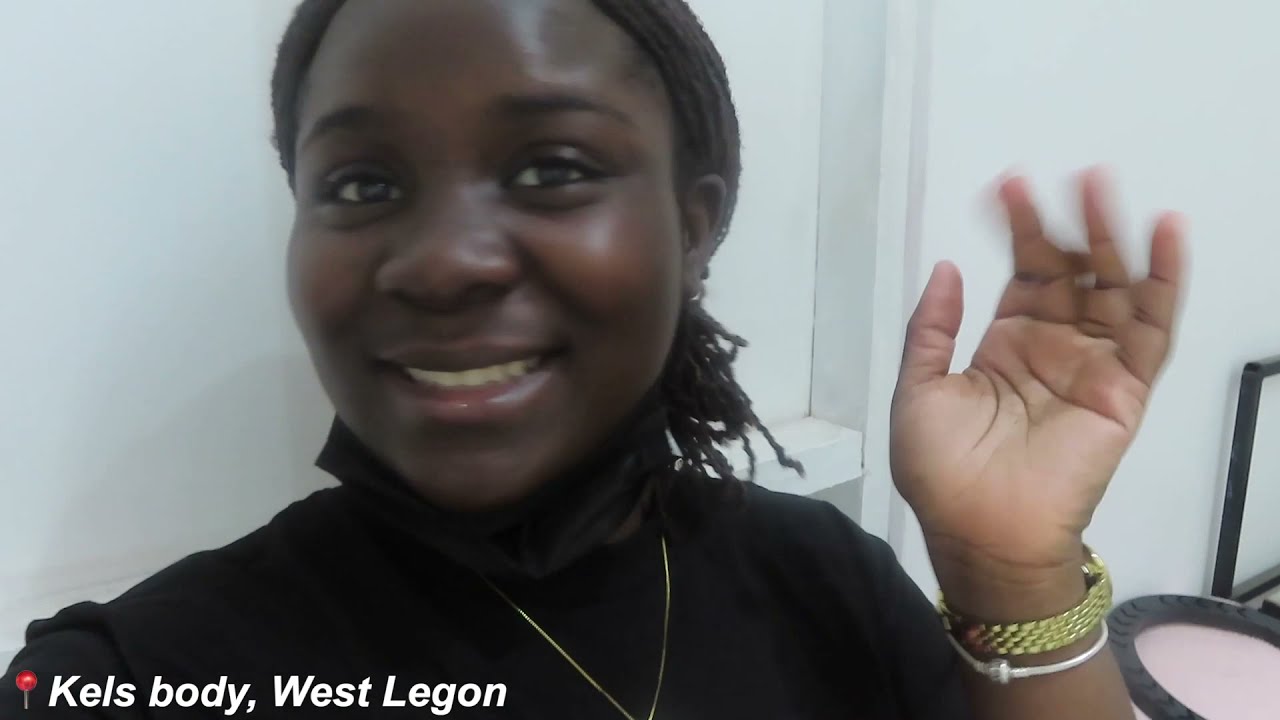The image features a smiling black woman with black braids and brown eyes, posing against a white wall. She is seen from the torso up, wearing a black shirt and a gold chain around her neck. Her left hand is raised as she waves, adorned with a gold watch and a silver bracelet. Her fingers appear slightly blurry, captured mid-motion. In the bottom left corner of the picture, there is a location pin icon followed by the text "Kel's Body, West Lagon." The background includes a small white shelf partway down the wall and a circular object in the bottom right-hand corner of the image.